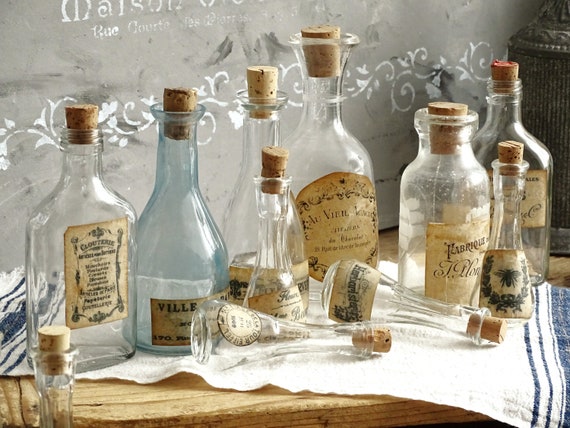The image features a collection of vintage-style glass bottles with cork stoppers, meticulously arranged on a wooden surface. These bottles, mostly clear except one with a smoky gray-blue tint, are beautifully labeled with yellowed paper adorned with intricate French text and decorative elements, such as a bee encircled by a floral wreath. Out of the ten bottles, eight stand upright while two lie on their sides. All the bottles are clearly empty. The bottles rest on a white dish towel with blue lines framing the left and right edges, enhancing the rustic charm of the setup. Behind the bottles, a gray wall embellished with white filigree designs and some indistinct French writing, along with an enigmatic metal decoration in the upper right corner, adds an artistic background to the scene.